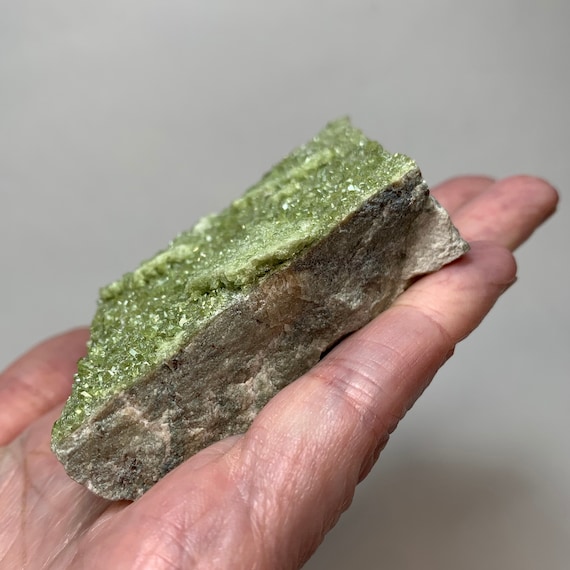This is a detailed close-up image of a man's left hand with the palm facing upward against a gray background, positioned from the bottom left to the top right corner at a 45-degree angle. The palm is held flat with straight fingers, each angled towards the two o'clock position. The man is holding a trapezoidal, finger-length specimen of an unrefined mineral or gemstone rock. The top of the rock showcases a vivid lime green surface adorned with smaller, crystalline structures and intersected by white veins. The rock's sides appear grayer and tanner, reflecting its raw, natural state. The rock has clearly been cut and cleaned, displaying the distinct layers and textures within, like green mineral sections and striated areas, evocative of a cold, squarish slab of stone.